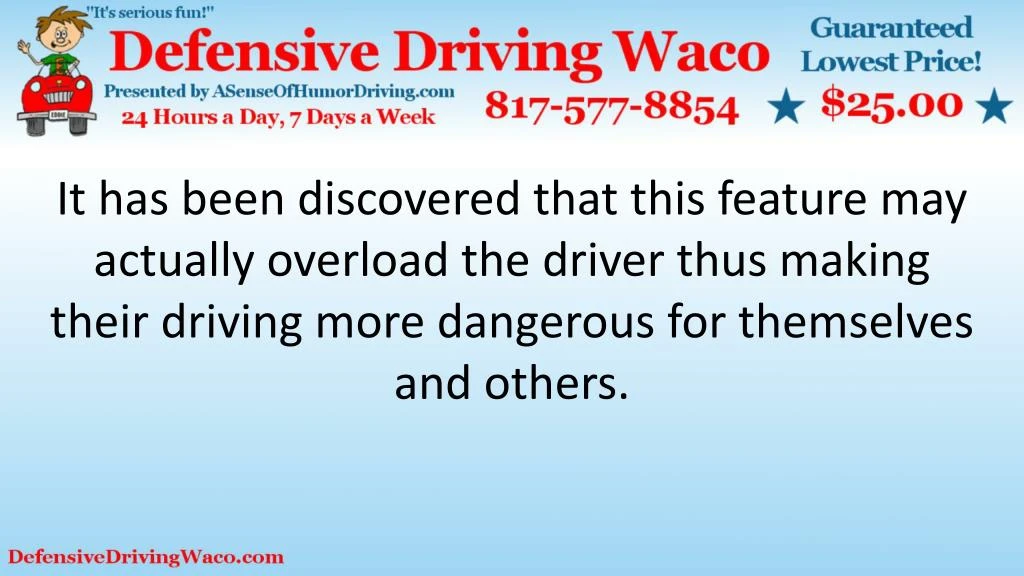This business card-shaped image promotes a defensive driving course in Waco, featuring prominent details in both text and graphics. At the top, in red text, it states "Defensive Driving Waco," accompanied by a cartoon boy in a red car. To the right, in blue font flanked by two blue stars, it declares "Guaranteed Lowest Price $25." Below the main heading, it says "Presented by Asenseofhumordriving.com," offering services "24 hours a day, 7 days a week," along with a phone number. The center of the image, in large black sans serif font on a bright blue background, warns: "It has been discovered that this feature may actually overload the driver thus making their driving more dangerous for themselves and others." At the bottom left, the URL "DefensiveDrivingWaco.com" is displayed, directing viewers to their website for more information.